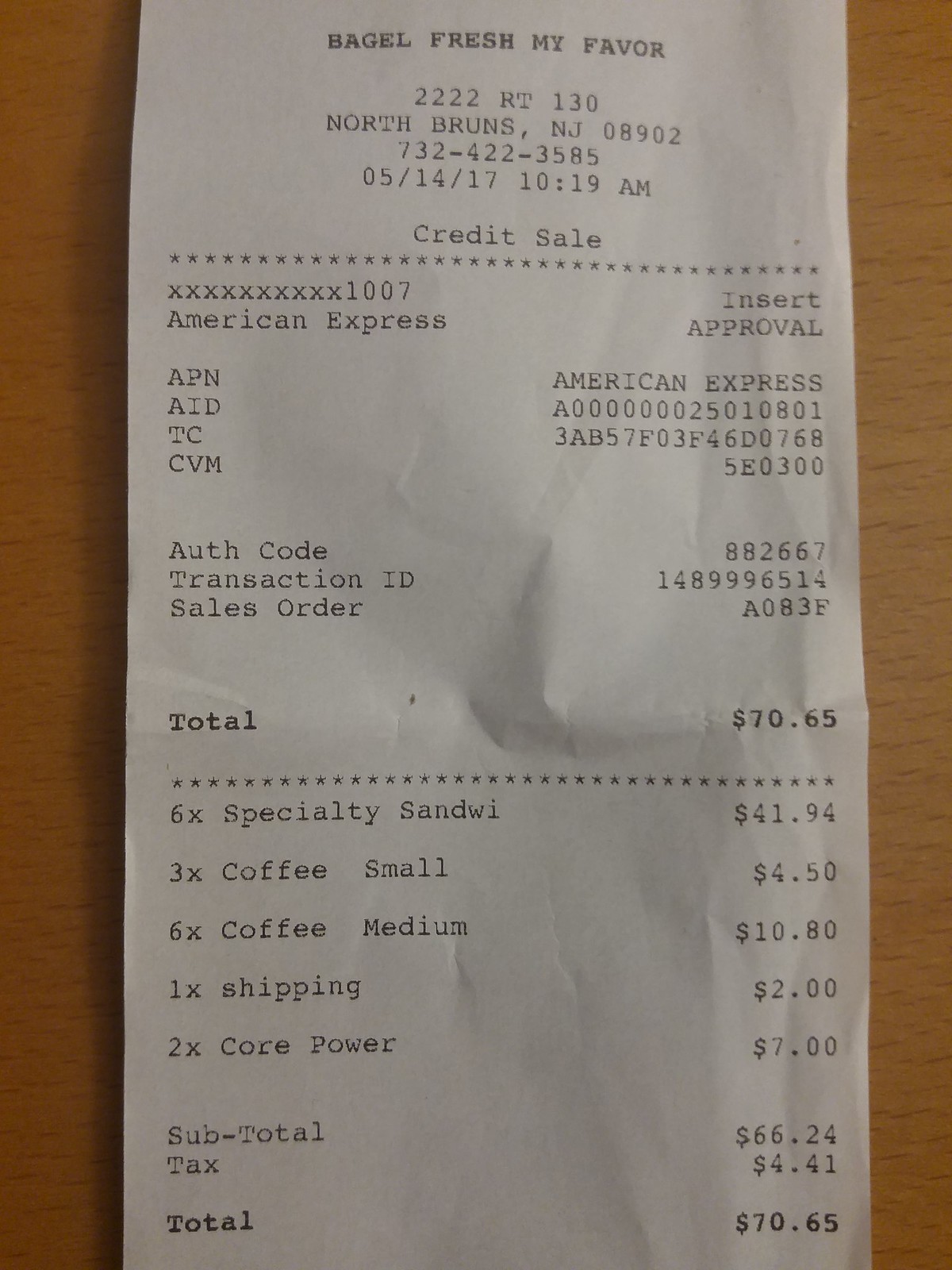This close-up photograph captures the details of a paper-white receipt. The backdrop features a light honey-colored wood grain surface, which adds a warm, natural tone to the composition. The zoomed-in view clearly showcases the printed information in black ink on the receipt. 

At the top, the receipt prominently displays the establishment's name in bold lettering: "Bagel Fresh My Favor". Directly beneath, the address "222 Route 130, North Brunswick, New Jersey 08902" is listed, followed by the contact phone number "732-422-3585".

The receipt also indicates the date "05-14-17" and the time "10:09:18 AM". Further down, it notes the payment method as a "Credit Sale" via "American Express." The total amount for the transaction is a surprisingly high $70, suggesting a substantial purchase, likely involving a significant quantity of bagels.